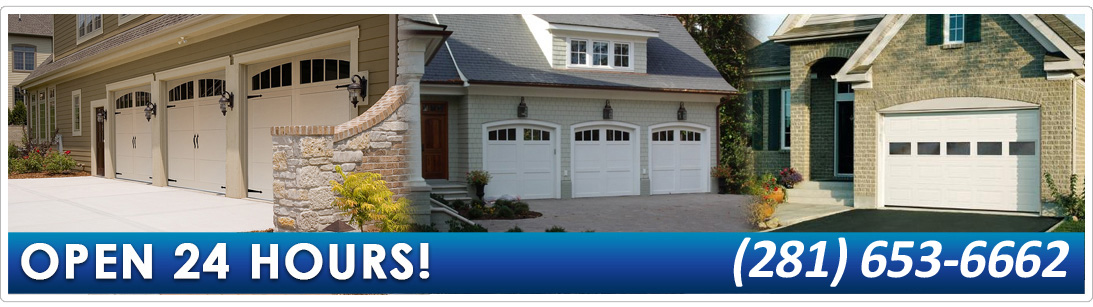This small banner ad prominently displays three houses available for sale, vacation rentals, or long-term rentals. The ad itself is compact, mostly dedicated to showcasing the homes with minimal text. 

The visuals on the banner are seamlessly edited so the images of the houses blend smoothly into each other without any hard edges. 

The first house on the left features a beige exterior and boasts three garages. The middle house also has three garages and is painted a light gray color. The third house on the right is a smaller, single-level house with a beige brick facade and a single garage. Each house is accompanied by an asphalt driveway, enhancing the uniformity of the presentation.

At the bottom right corner of the ad, the phrase "OPEN 24 HOURS" is prominently displayed in all capital letters. Conversely, the bottom left corner contains a contact phone number: 281-653-6662, inviting viewers to inquire further about the properties.